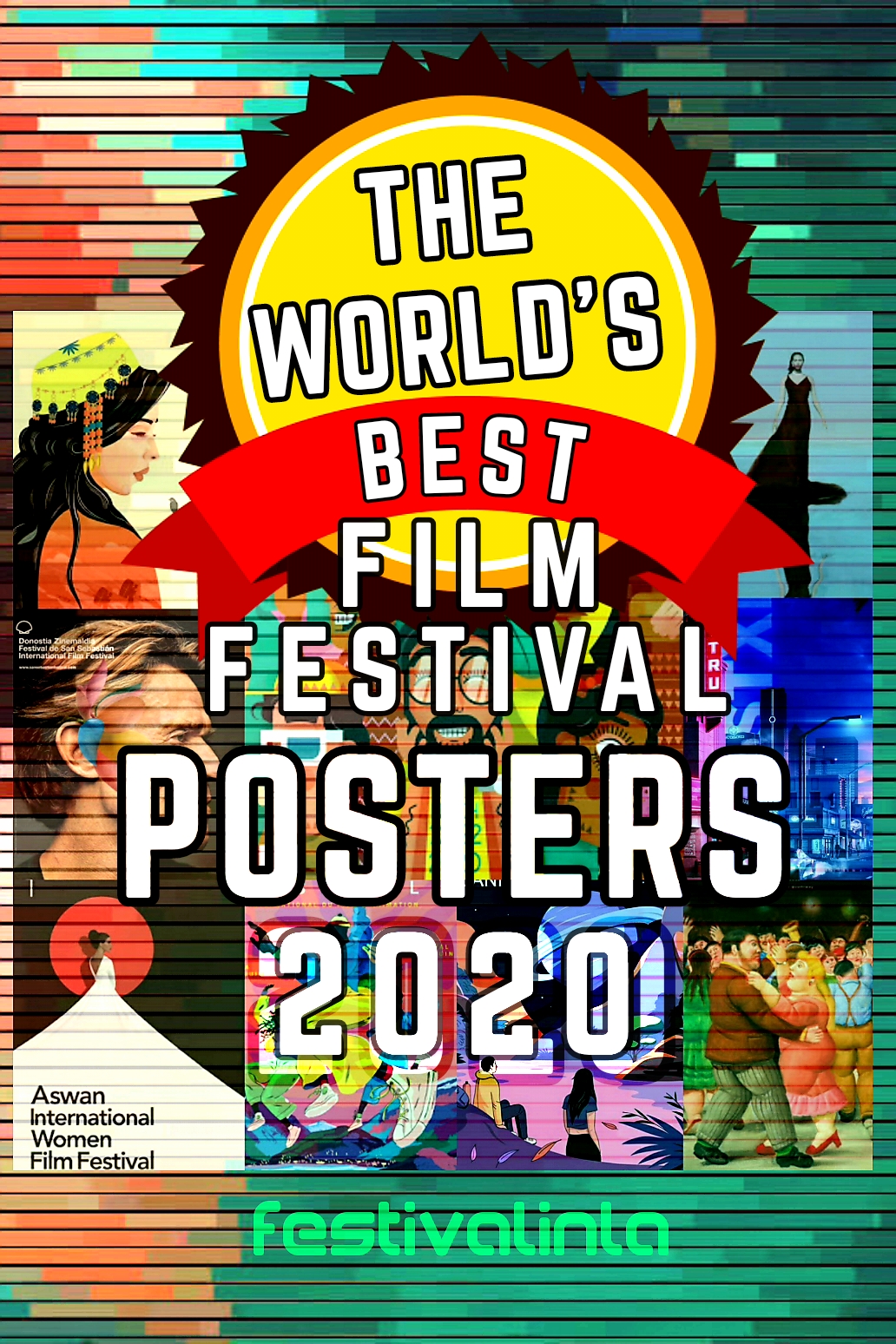This vibrant and colorful promotional graphic showcases "The World's Best Film Festival Posters 2020" in bold white text with a black outline, positioned prominently in the center. The text "best" is superimposed on a red ribbon that crosses a yellow circle with a jagged black border. The background features a greenish, horizontal wood slat texture, subtly showing through a diverse collage of movie posters and animated images, including notable ones like a cartoon of a man dancing with a woman, surrounded by people. Hints of pink, red, green, and blue add to the vibrant array of colors, making the image eye-catching and dynamic. At the bottom, semi-transparent green text reads "Festival Inla," potentially indicating the media outlet or organizer behind this vivid promotional piece. This image, likely used online or on social media, effectively highlights the creativity and variety of film festival posters.